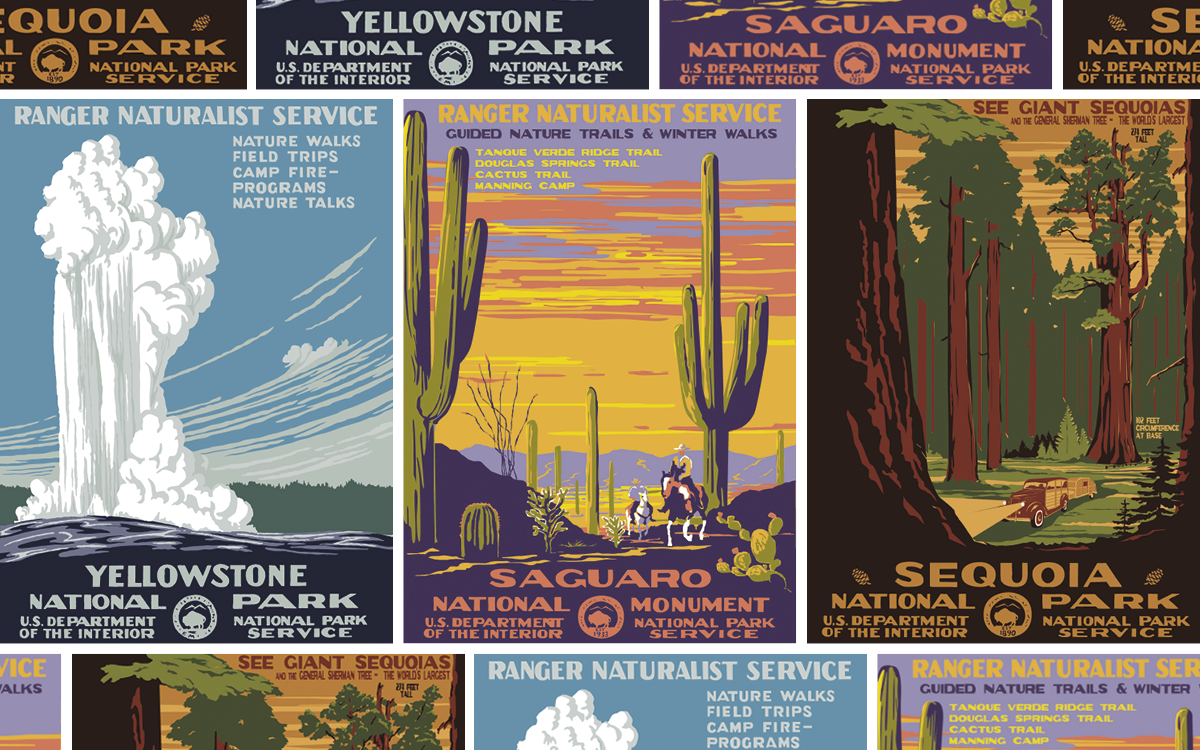This image features a visually captivating collage of nine vintage-style posters, prominently displaying three iconic national parks: Yellowstone, Saguaro, and Sequoia. Arranged in a rectangular landscape format, the collage consists of four rows, with the middle row occupying about 70-75% of the image's central space. This central row showcases full posters for each park.

On the left, the Yellowstone National Park poster commands attention with a striking white geyser, likely Old Faithful, set against a primarily blue backdrop that transitions from light to dark. The middle poster for Saguaro National Monument bursts with desert colors, showcasing cacti and two horseback riders moving along a purple-hued path under an orange sky. The rightmost poster highlights the towering Sequoia trees, where a classic car pulling a trailer is depicted driving through the verdant scene. Each poster's text includes the U.S. Department of the Interior on the left and National Park Service on the right.

The top and bottom rows add to the collage's retro aesthetic by repeating portions of the central posters. The top row features the bottom sections of the Yellowstone, Saguaro, and Sequoia posters, highlighting their titles, while the bottom row shows the upper parts, such as the geyser in Yellowstone, the desert scene in Saguaro, and the towering trees in Sequoia. The overall color scheme includes vibrant greens, blues, yellows, and purples, contributing to the nostalgic, vintage feel of the collage, further enhanced by the intricate and colorful details of each park's unique landscape.